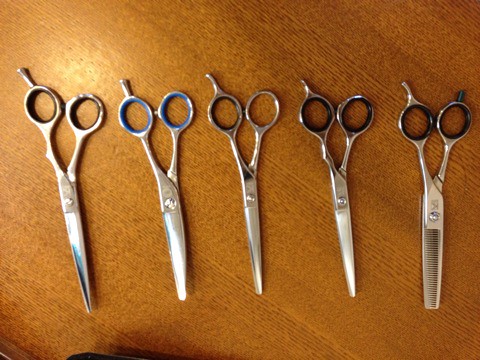The image depicts five pairs of shiny, stainless steel hair-cutting scissors laid out side by side on a burnt orange-colored wooden table. Each pair has finger loops positioned upwards with single screws securing the blades together. Notably, the second pair from the left features blue-colored finger loops, while the loops on the two pairs to its right are black. The rightmost pair of scissors is distinct, featuring comb-like blades designed for thinning hair. The remaining scissors all have standard pointed blades, reflecting high polish and craftsmanship.